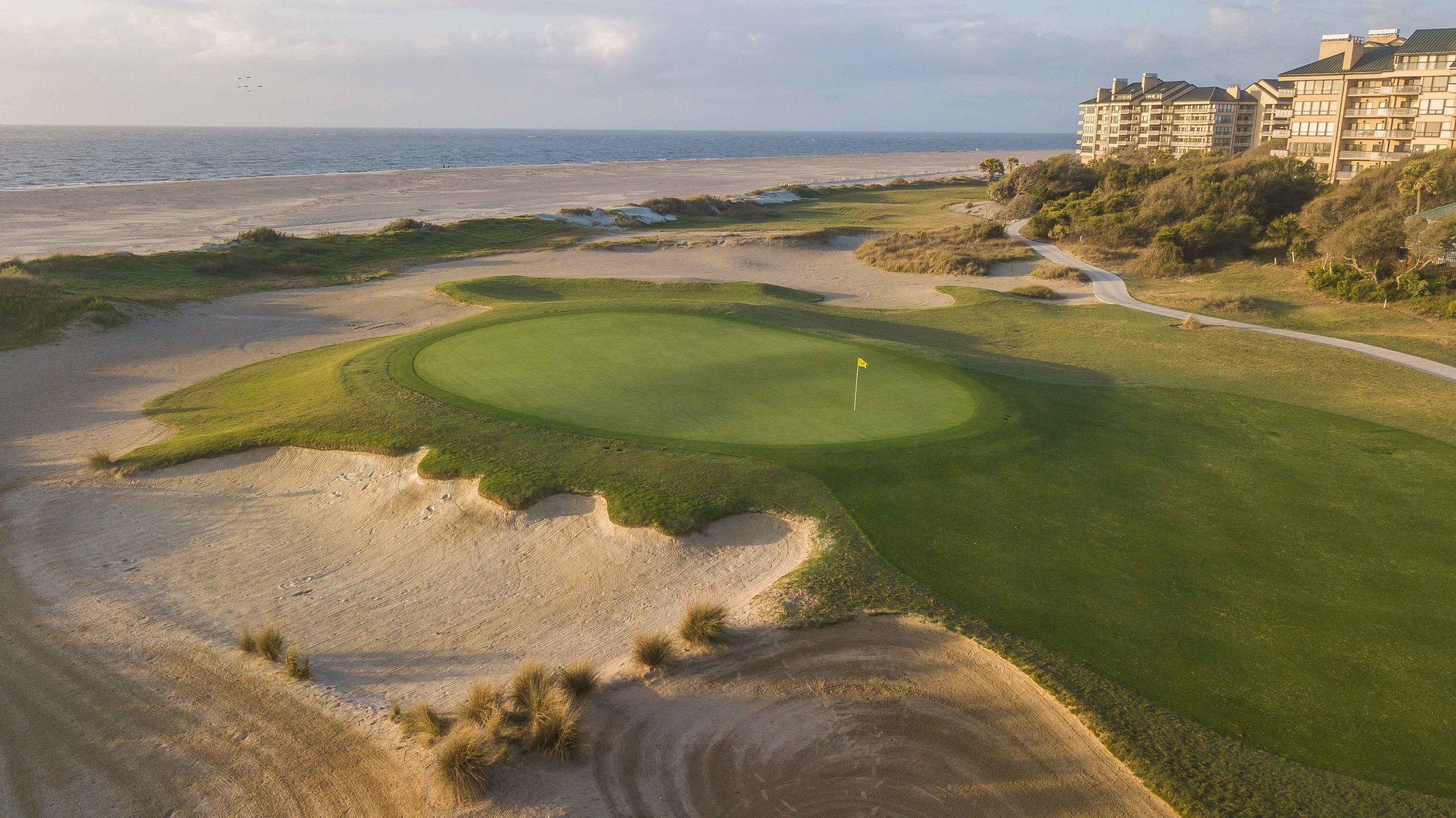The image captures an aerial view of a picturesque golf course set against a coastal backdrop. In the foreground, there's a meticulously maintained grassy area featuring a prominent circular platform with a yellow flag on a tall pole marking one specific hole. Surrounding this elevated green circle is darker grass, which contrasts sharply with the expansive sand dune encircling three-quarters of it, reminiscent of a sand hazard typical on golf courses. Just beyond this sandy expanse, we observe a wide beach leading to a large body of water, likely the sea, dominating the upper portion of the image.

To the right of the golf course, a road snakes along, bordered by a dense cluster of trees. Further right, there’s a collection of several tall buildings, presumably apartments or hotels, ranging from four to seven stories, featuring numerous windows and balconies. These buildings stand out against the clear blue sky, which is dotted with a few scattered white clouds, completing the serene coastal landscape that integrates both natural and urban elements.